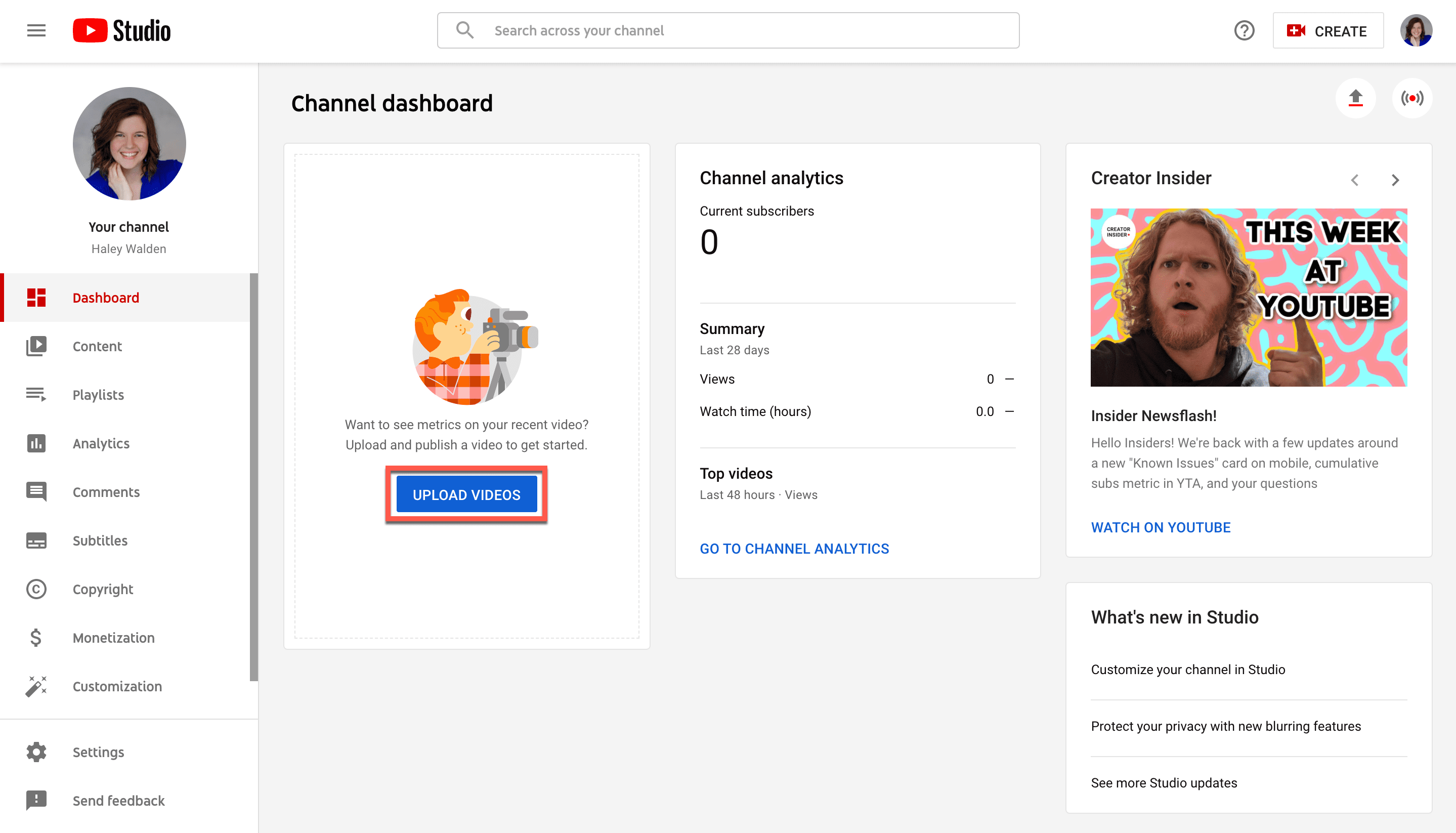In the image, we see a detailed snapshot of a YouTube Studio page belonging to a user named Haley Walden. At the top left corner of the interface, the familiar YouTube logo and the word "Studio" are displayed on a white background. Below the logo, three horizontal lines, typically used to access menu options, are visible. To the immediate right of the site's name, a white search box with the placeholder text "Search across your channel" invites users to find specific content on their channel. Adjacent to the search box is a black-outlined circle with a black question mark, providing access to additional information and support.

Next to the help icon, there's a white box with a red and white camcorder icon and the word "Create" in black, indicating content creation options. Further to the right, Haley's account icon personalizes the page. Below the top navigation area, on the left sidebar, Haley's account icon is again displayed along with the words "Your channel" and her name "Haley Walden."

The sidebar lists various categories such as Dashboard, Content, Playlists, Analytics, Comments, Subtitles, Copyright, Monetization, Customization, Settings, and Send feedback. The Dashboard category is highlighted in red, showing that it is currently selected, while the remaining categories are in gray.

The main focus of the image is the channel dashboard itself, which is divided into four distinct sections. The first section on the left contains a blue button labeled "Upload Videos," outlined in red, ready for content uploads. The middle section, titled "Channel Analytics," displays the current number of subscribers, a summary of the channel’s performance, and top videos with a blue link prompting users to go to channel analytics for detailed insights.

On the right side, there are two more sections. The top one, "Creator Insider," offers updates on YouTube’s latest activities and features a blue link to watch more on YouTube. The bottom section, "What's New in Studio," lists recent updates to the Studio, with an option to see more detailed updates.

This structured layout provides a comprehensive overview of Haley Walden's YouTube channel management tools, blending functionality and ease of access.